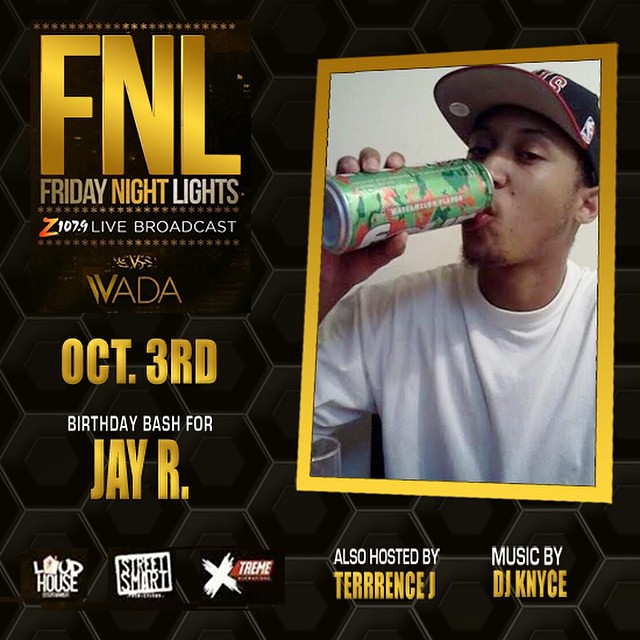The promotional flyer features a sleek, dark honeycomb-patterned background with a sophisticated gold-black color scheme. On the top left side, bold, gold letters read "FNL" and just below, "Friday Night Lights" followed by "Z107.9 Live Broadcast." Hovering above and below these titles are decorative rows of stars. The flyer details an event on October 3rd, labeled as a "birthday bash for JR," with "WADA" written prominently. The right side of the flyer showcases a young black man, presumed to be JR, wearing a white shirt and a Chicago Bulls hat. He is drinking from a large green and orange can of Four Loko, looking straight at the camera. The bottom of the flyer highlights additional hosts, noting it is "also hosted by Terrence J" with "music by DJ K-Nice." The footer features logos representing multiple comedy scenes, adding to the event's festive nature.